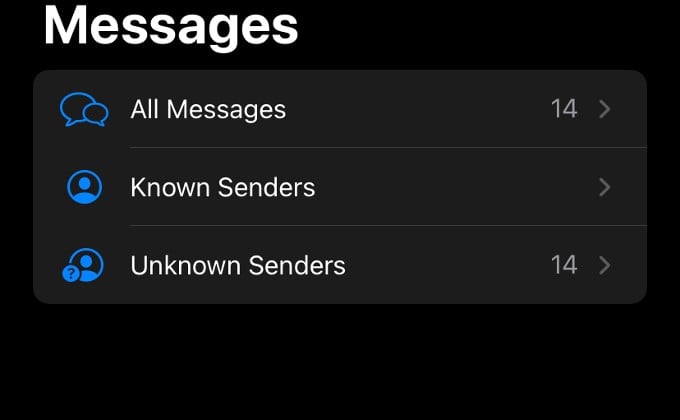The image depicts a black-background messages window interface. At the top left corner, there is a prominent, white-colored title "Messages" with an uppercase 'M' followed by lowercase letters. In the center of the screen, a grey rectangle with rounded edges is divided into three sections.

The upper section is titled "All Messages," with the 'A' in "All" and the 'M' in "Messages" capitalized. It shows the number 14 next to a small arrow for expansion. Below this is the "Known Senders" section, with 'K' in "Known" and 'S' in "Senders" capitalized. This section has an expandable arrow but no listed items. The bottom section is labeled "Unknown Senders," featuring an uppercase 'U' and 'S', also showing the number 14 next to an expandable arrow.

Each section is accompanied by a blue icon on the left. For "All Messages," the icon consists of two overlapping, empty speech bubbles. The "Known Senders" icon is a circle enclosing a stylized head and torso. For "Unknown Senders," the icon mirrors the "Known Senders" symbol but includes a small question mark to the left of the figure.